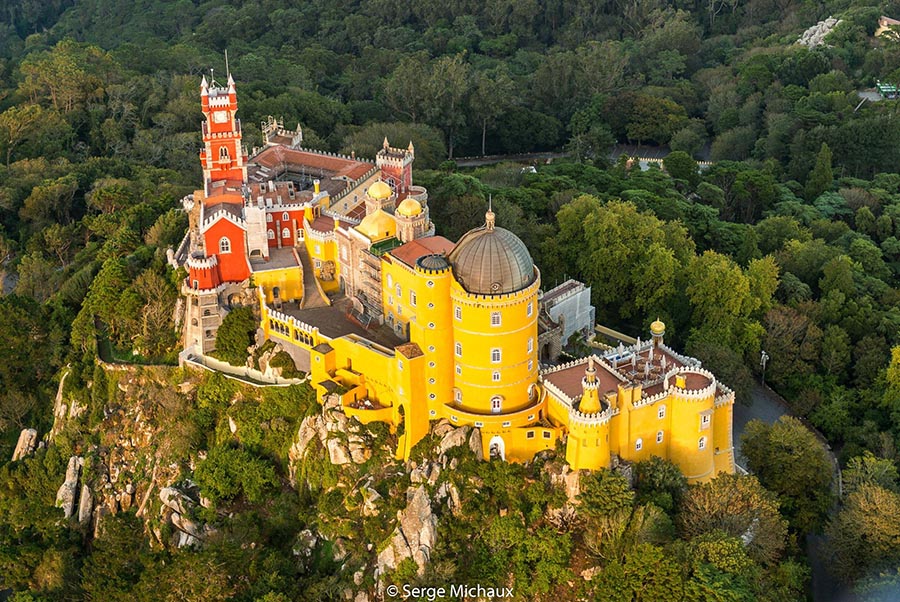This aerial, bird's-eye view presents a vivid and sprawling image of a castle complex majestically perched on a hill or mountain. The castle features distinct sections: the front part is bathed in a golden yellow, while the back part showcases a bold orange hue with white trim. Multiple structures such as rectangular buildings, cylindrical towers, and golden domes with circular gold furnishings crown various rooftops, adding to its grandeur. White fences also adorn parts of the roofs. The castle's intricate architecture is complemented by its surrounding environment; lush green trees and shrubs blanket the rocky outcropping on which the castle stands. Beyond the hill, dense forest continues, punctuated by visible roadways or pathways cutting through the greenery towards the upper right and bottom right of the image. The overall setting conjures up a serene and picturesque landscape, reminiscent of something found in the Swiss countryside.